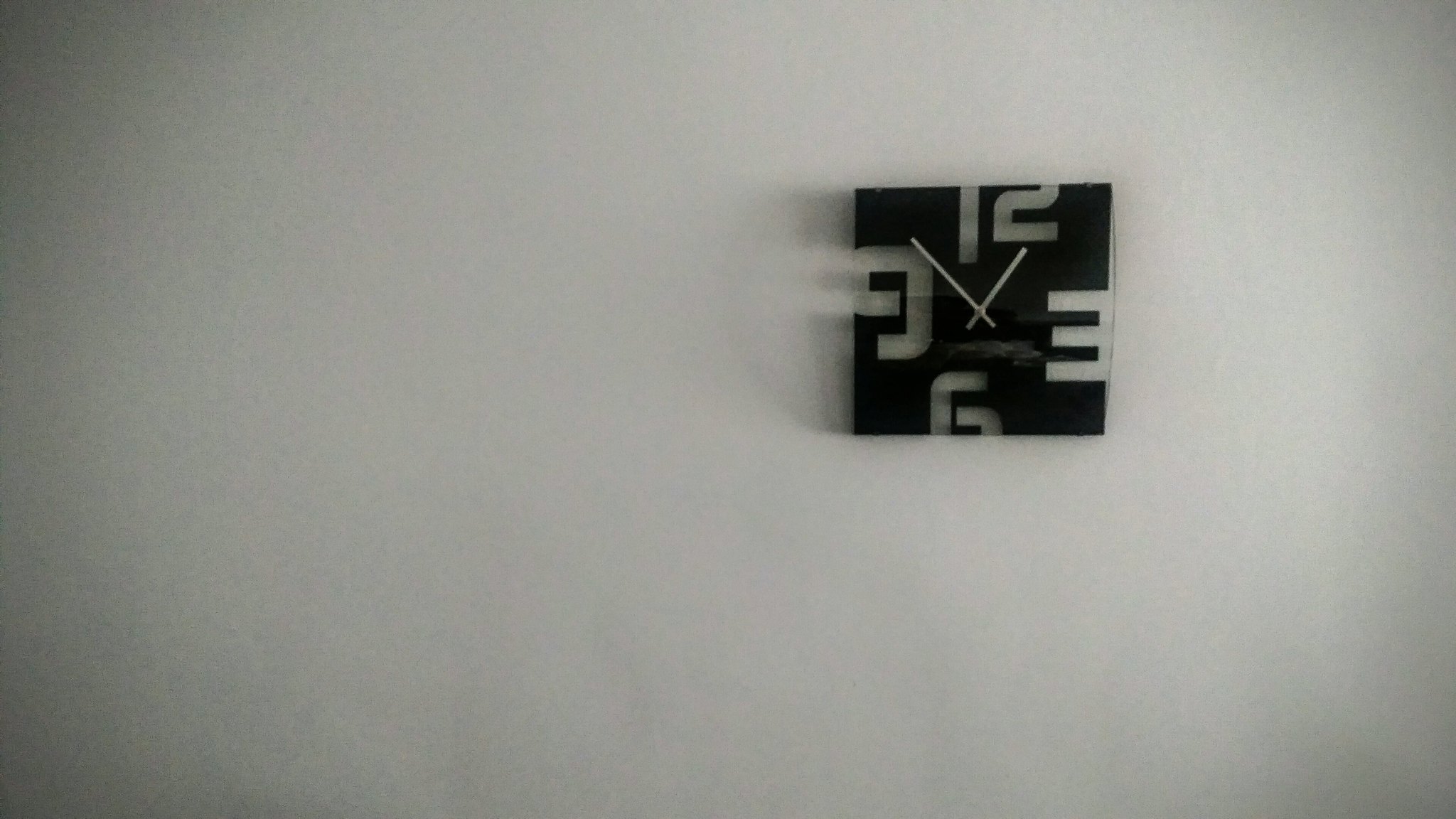This is a digital photo in landscape orientation with a predominantly white background that exhibits inconsistent lighting, casting shadows around the edges. The focal point, just past the center towards the right, is a modern-style black square clock. Intricately designed, the clock features large numerals—12, 3, 6, and 9—strategically cut out of the black square, giving an open space effect. The material appears to be either black glass or plastic, lending it a sleek and contemporary aesthetic. The clock has white hands, showing the time as approximately twelve-fifty, or ten minutes to one.